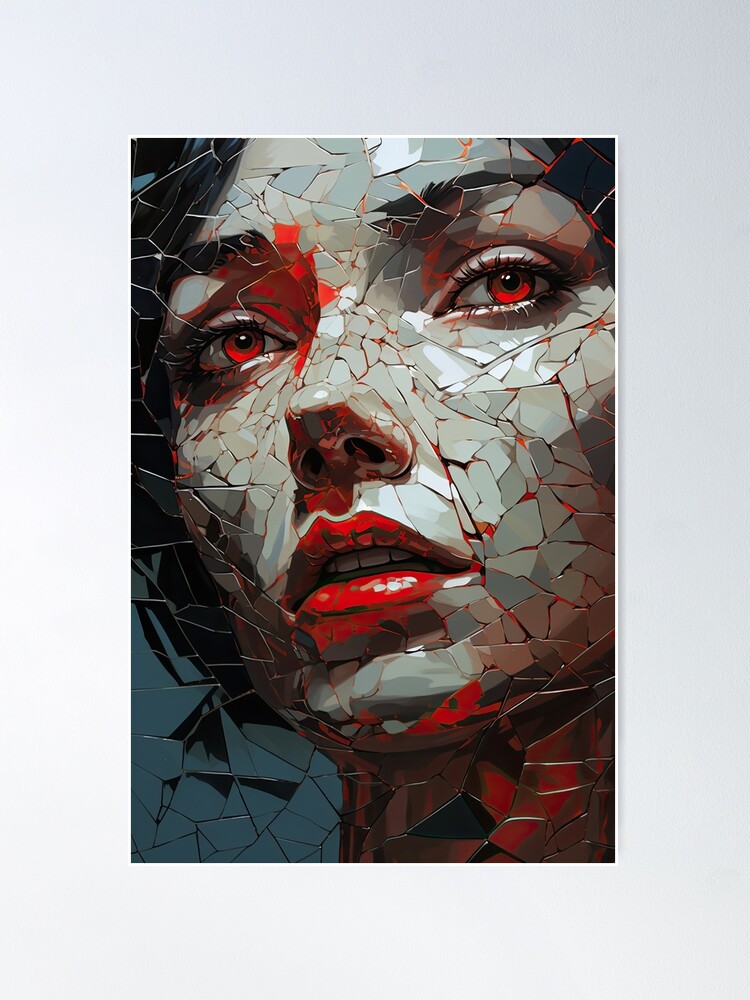The detailed image depicts an artistic rendering of a woman's face in close-up, capturing her profile from the neck up. The portrait, possibly a painting, showcases her grayish, almost white complexion with striking bright red accents. Her eyes are a vivid red, with a matching bright red lipstick, and there are red shadows and highlights around her eye and chin, contributing to the overall haunting aesthetic. The woman's hair is black, and the painting's overall tone is cool, featuring dark black and steel blue hues. The artwork is fragmented, resembling tiny broken tiles or shards, creating an effect of a face cracked and shattered into pieces. The background and cracks are also imbued with red, deepening the intensity of the image. The woman appears to be looking slightly to the right, away from the viewer. There's a sense of realism in the rendering of her eyes compared to the rest of the image, and the piece exudes a sense of a mural or a surface that either has naturally cracked or deliberately designed to appear fragmented.